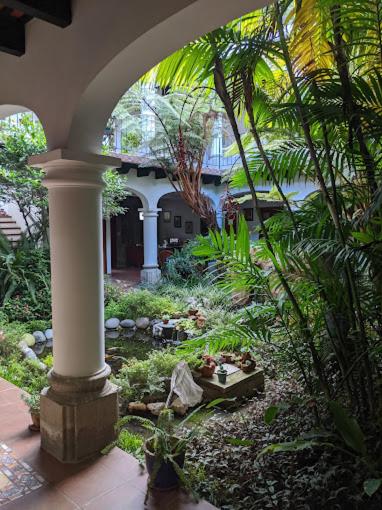This image captures a luxurious villa with royal architecture, characterized by its grand white pillars and expansive verandah. The exterior of the building glistens in white, underlined by elegant arched openings. The verandah overlooks a well-maintained garden teeming with diverse plant life. The garden features various ferns, bushes, and leaves that partially conceal the villa's structural beauty. A small water body, adorned with surrounding rocks and pebbles, adds tranquility to the lush scene. A wooden box with clay items rests beside this serene pond. The flooring of the verandah is composed of reddish-brown tiles, complementing the grandeur of the place. In the background, more rooms are visible, embellished with photo frames and furnished with tables and chairs, although they are largely hidden by the vibrant green foliage. Sunlight filters through the leaves, giving a daytime shimmer to the verdant surroundings and highlighting the architectural splendor of the villa.